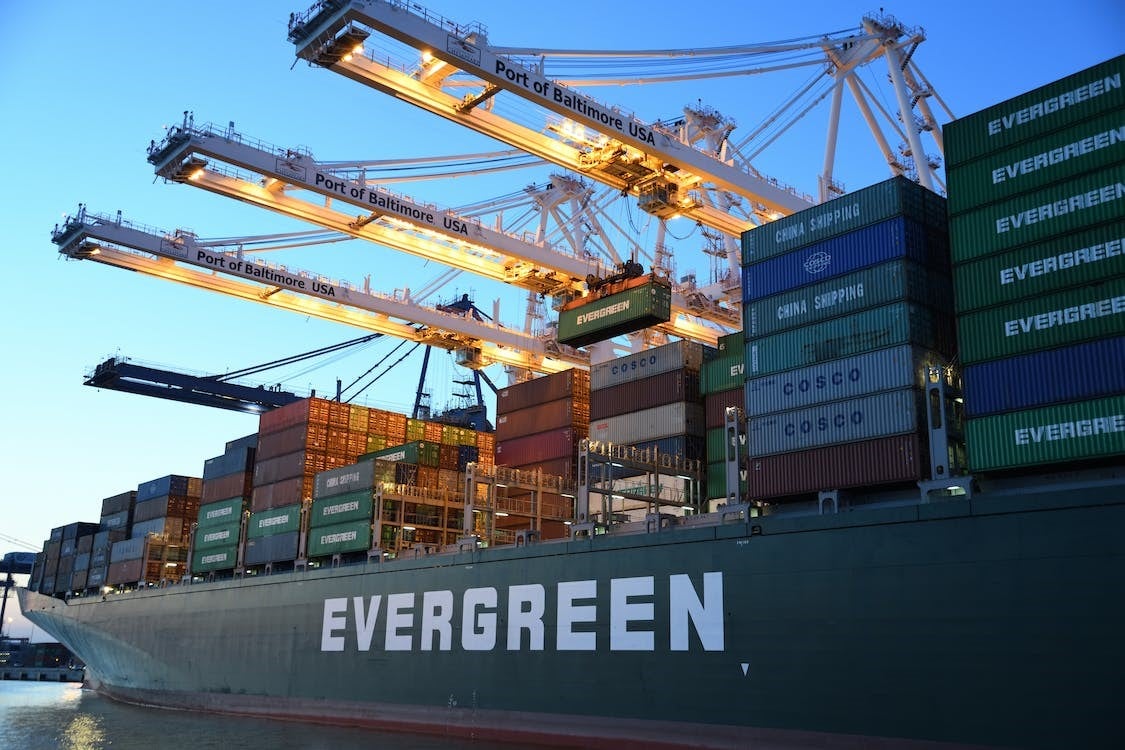This color photograph captures an extremely large, green container ship with "Evergreen" prominently displayed in bold, white capital letters along its side. The ship is floating in a body of water and is stacked high with hundreds of cargo containers in various colors—green containers with "Evergreen," white containers with "COSCO" in blue, and other containers marked "China Shipping" in white letters. Additional containers come in shades of blue, gray, and red. There are four massive cranes over the ship, all labeled "Port of Baltimore USA" in black letters. The crane to the right is actively lowering a container, integrating it into the meticulously arranged rows of cargo. Strings of lights and additional structural features can be seen hanging above the ship, adding to its complex and industrious appearance, but no people are visible in the image.